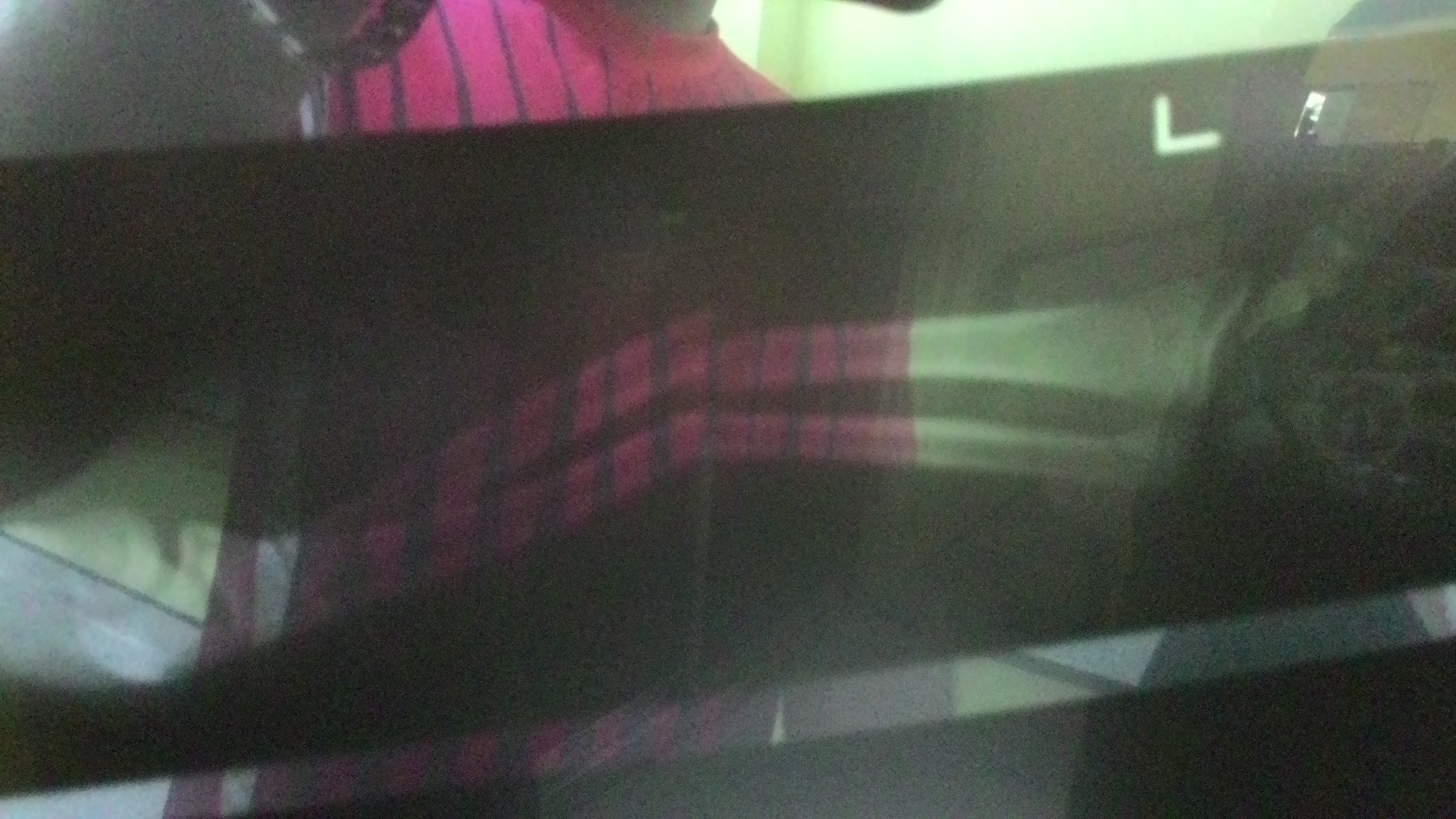The photograph presents an abstract and somewhat enigmatic scene featuring a person whose gender is ambiguous. They are wearing a bright pink and black striped garment that appears to be a very short t-shirt or skirt. The person is standing behind a translucent black object, which resembles an x-ray display showing the fractured bones of an arm. This x-ray, either behind glass or integrated into a pane, obscures parts of the person's body, making identification challenging. The background of the image is dominated by diffused light, possibly green, and appears murky, hinting at a setting reminiscent of a nightclub or a dark, gothy environment. There might be additional objects in the backdrop, such as a bed and a pillow, adding to the uncanny ambiance of this abstract visual composition.